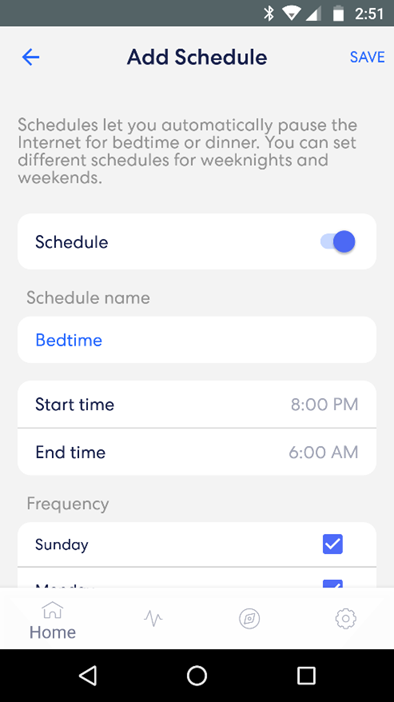This screenshot displays a scheduling application on a mobile phone. At the very top, there's a gray border featuring several icons: a Bluetooth icon, a Wi-Fi icon, a data connection icon, and a nearly full battery indicator, with the time displayed as 2:51. Below this top border, within a gray background area, there's a blue left-pointing arrow symbolizing the back function, "Add Schedule" centered in the middle, and "Save" located in the upper right corner.

The main section of the screen highlights information explaining that schedules allow automatic pausing of the internet before bedtime or dinner. There's a toggle switch for enabling or disabling the schedule, which is currently blue, indicating it's active. The schedule is named "Bedtime," also shown in blue, with a start time set for 8 p.m. and an end time for 6 a.m. The frequency section shows checkmarks for Sunday and Monday, although the remaining days get cut off in the image.

At the very bottom of the screen, there's a black navigation bar containing several icons: a back arrow, a home button, and an icon for opening other tabs/apps. Additionally, just above this bar are app-specific icons including a home icon, a lifeline-style icon, a GPS icon, and a cogwheel icon, presumably for settings.